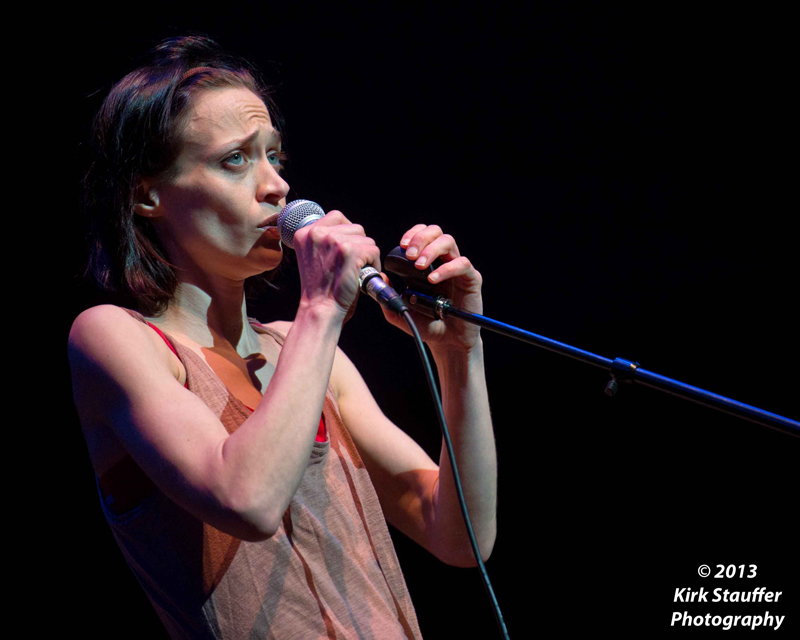The image depicts a thin Caucasian woman on stage, illuminated by spotlights from the bottom right corner, set against a solid black background. She has short dark hair and blue eyes. She is passionately singing into a silver microphone with a black cord, which she holds in her right hand. Her left hand grips the blue metal microphone stand. Her facial expression is intense, with a scrunched forehead and slightly sunken cheeks. She is wearing a peach and black tank top, possibly layered over a red tee, revealing her bare arms. The text “© 2013, Kirk Stauffer Photography” is visible in the image.